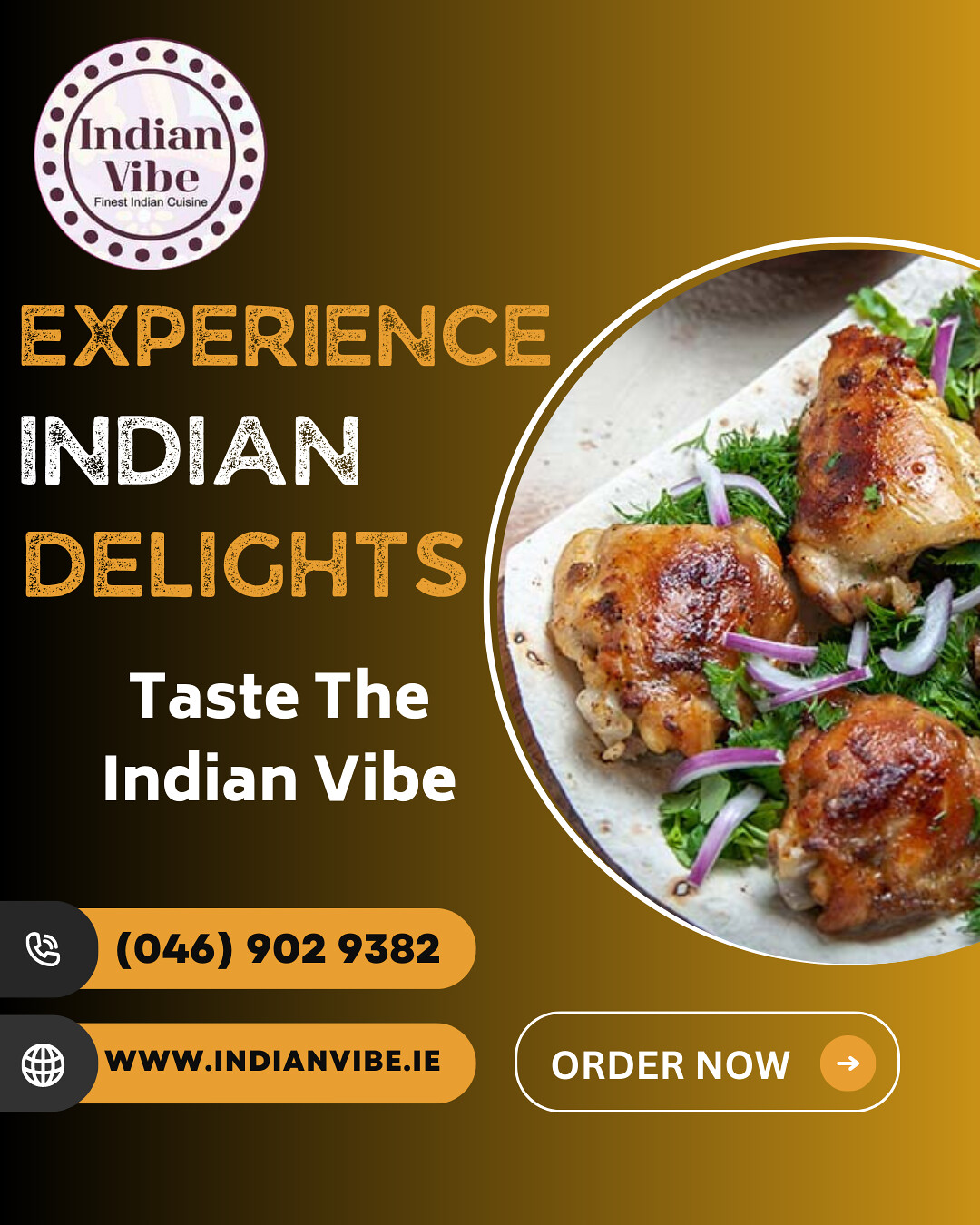This is an advertisement for Indian Vibe, Finest Indian Cuisine, featuring a warm brown background that transitions to gold towards the right side. At the top of the ad, there's a white circle resembling a plate, adorned with brown dots around its edge. Inside the circle, it reads "Indian Vibe. Finest Indian Cuisine." Below that, additional phrases like "Experience Indian Delights" and "Taste the Indian Vibe" are prominently displayed. 

Midway on the right side of the ad, there's an enticing image of a delicious dish: nicely browned chicken thighs accompanied by sliced purple onions and a bed of vibrant green vegetables. The overall design includes several key details: a graphic of a phone icon alongside the number 046-902-9382, a planet icon next to the URL www.indianvibe.ie, and an arrow pointing towards a call to action reading "Order Now." The text is presented in a grunge font, using gold and white colors that complement the background, delivering a visually appealing and comprehensive advertisement for this Indian restaurant.